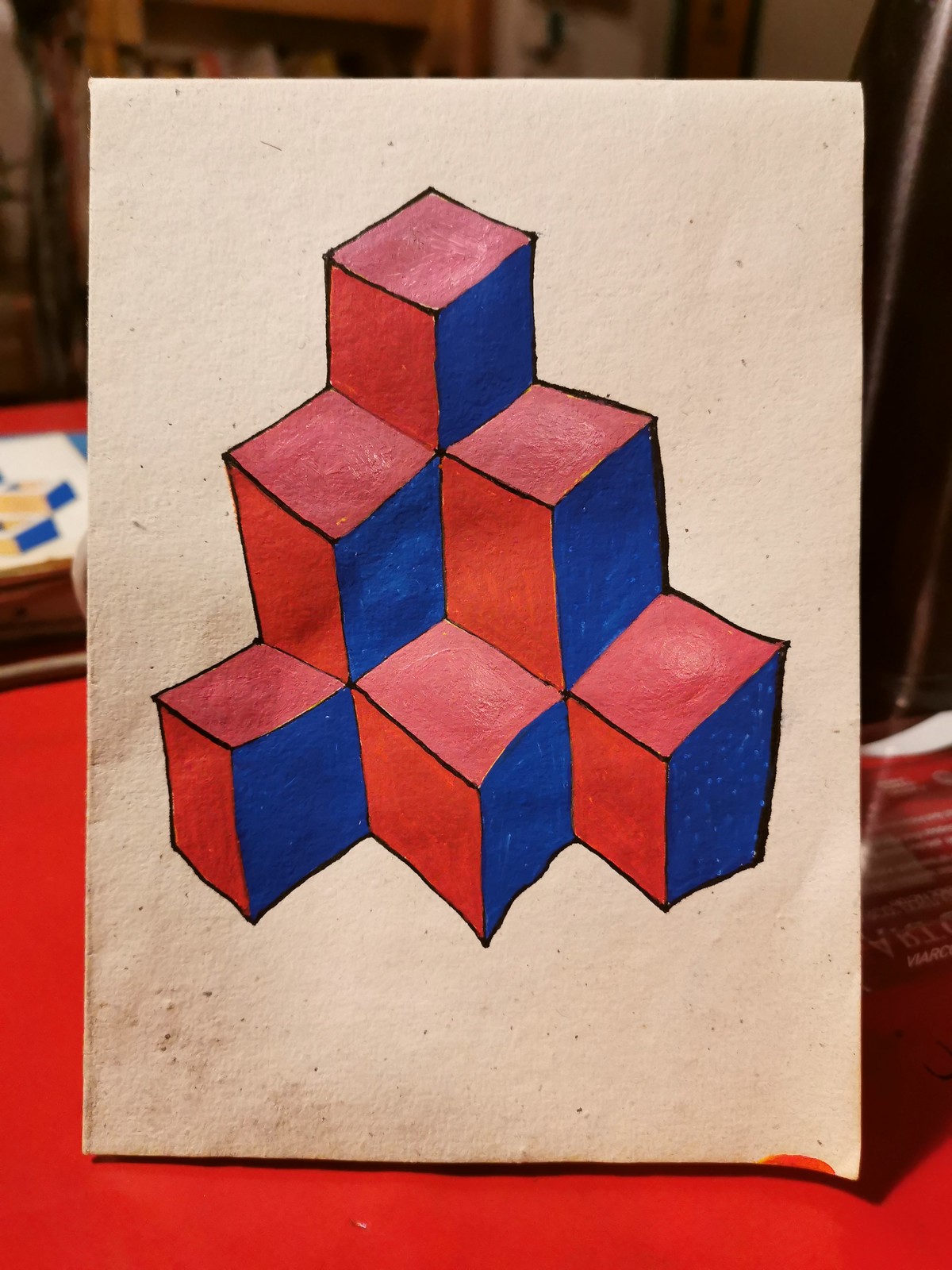A close-up photograph captures a white piece of paper standing vertically on a vibrant red table. At the heart of the paper, there is an intricate drawing of 3D blocks meticulously stacked in a pyramid formation: three at the base, two in the middle, and one on top. The detailed illustration reveals three visible sides of each block; the top and left sides are vividly colored red, while the right sides are shaded in blue, giving each block a striking blue face and red top and edges. Notably, the paper shows slight imperfections: the bottom left corner appears smudged with dirt, and the bottom right corner bears a small orange mark.